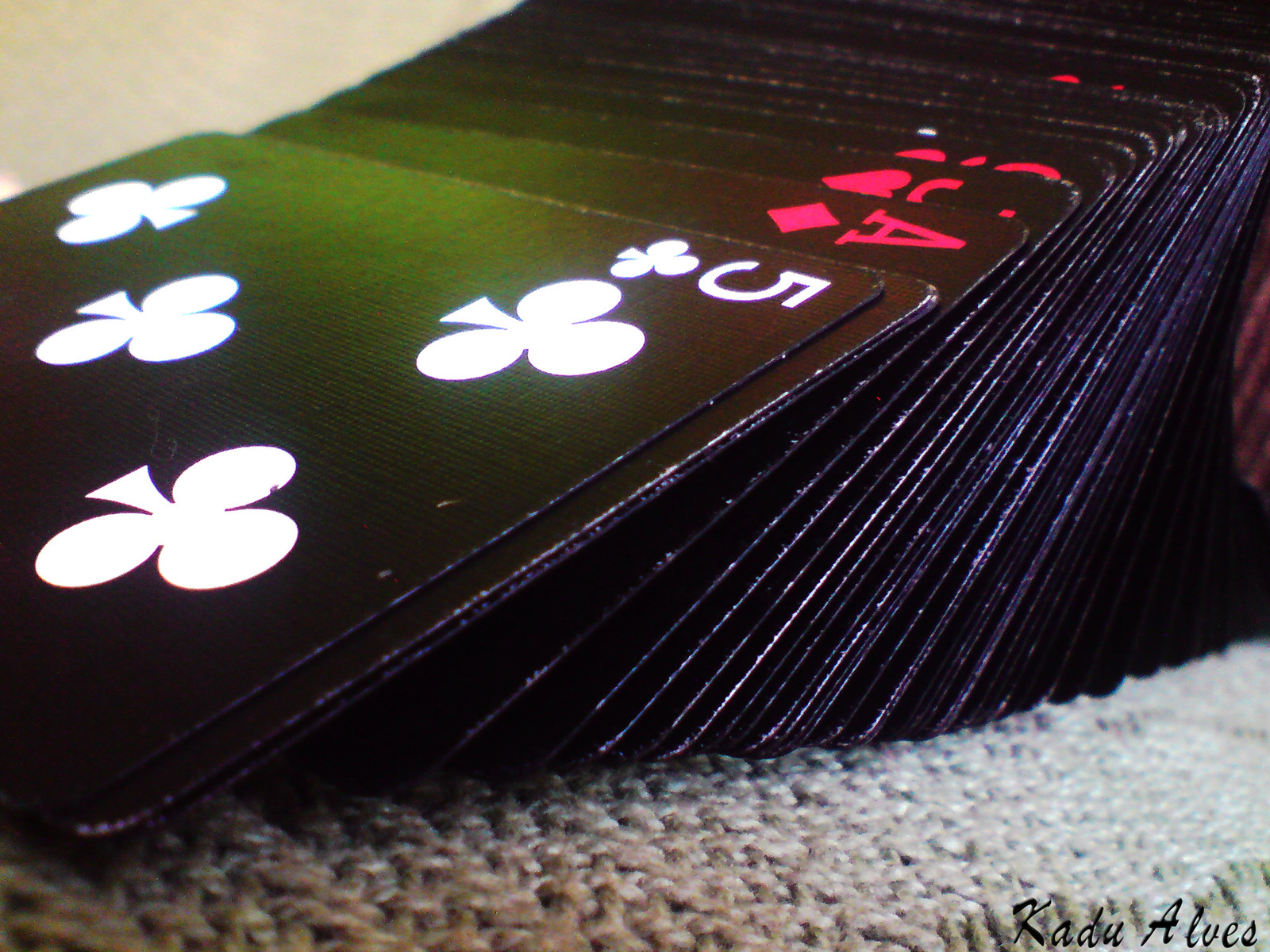The image showcases a collection of playing cards that resemble a standard 52-card French deck but are uniquely designed with an all-black background instead of the traditional white. These cards appear to be made from different materials, giving them a distinct look and feel. In the scene, there are approximately 20 to 30 cards being arranged into a deck. Unlike a typical deck, where cards are stacked flat on their backs, these cards are balanced precariously on their edges. The deck is positioned on some sort of material that provides support for this unusual arrangement. At the front of the deck, a five of clubs card is prominently visible. Behind it, various other cards, including an ace of diamonds, can be seen. Due to the black background, the suits of clubs and spades stand out in white, creating a striking contrast that accentuates the card designs.